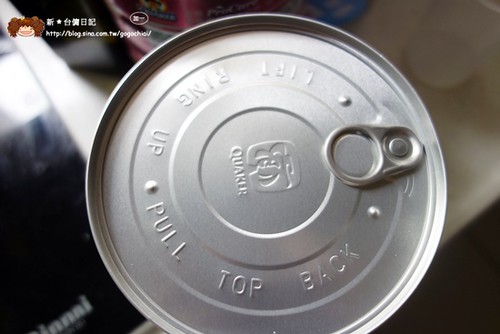This photograph captures the top of a silver can that features intricate details and various text elements. In the top left-hand corner of the can's lid, there is a vibrant illustration of a girl with large brown hair, next to which are characters that appear to be in Mandarin. Below the illustration, there is a web address: "http://blog.csite.com.tw/go/go", suggesting this image might be linked to someone's live blog or personal site. 

The can itself is metallic and has a distinct rim that slightly protrudes. There's a pull tab located on the left side of the lid. Just to the right of this tab, the can instructs users on how to open it with the text: "Pull to the bottom, pull top back and lift ring up." Additionally, there is a logo near these instructions that resembles a flower, accompanied by the brand name "Quaker."

The can is set on a beige countertop, and in the background, there are some miscellaneous objects, adding context and a sense of everyday environment to the scene.